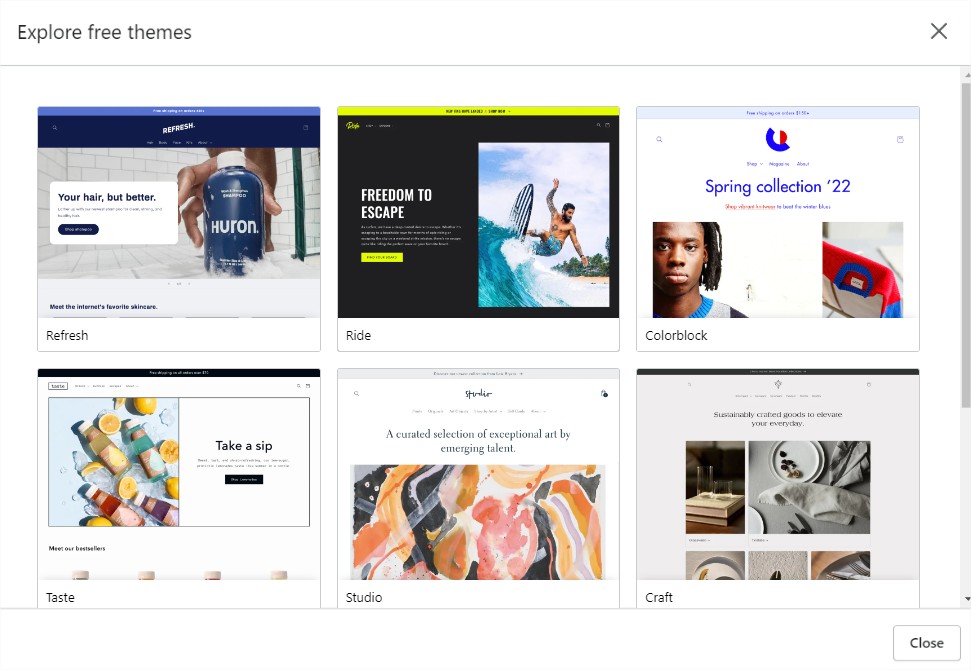In the image, there is a dynamic screen interface showcasing various thematic displays and interactive elements. At the top, a notification prompts users to "Explore Free Themes," which can be dismissed with an 'X' button. Below this notification, there is a section labeled "Your Air But Better," featuring a blue strip across the top and a darker black strip with a 'Refresh' button. Beneath this, several interactive options are available, including a button labeled "Your Hair But Better," which users can click for more details.

The scene also includes a person reaching towards the bottom of a shower stall to pick up a ball imprinted with the word "Huron." Adjacent text highlights "Meet the Internet's Favorite Skincare," accompanied by a 'Refresh' button.

Another section titled "Freedom to Escape" features an image of a surfer expertly riding a wave. The text "Ride" is prominently displayed, showcasing different styles with color blocks in red, white, and blue from the "Spring Collection 22."

On the right panel, a segment called "Taste" displays an assortment of colorful, fruit-infused drinks laid out on ice, inviting viewers with the phrase "Take a Sip." Further below, another section entitled "Studio" presents a modern art painting alongside a description of "A Curated Selection of Exceptional Art by Emerging Talent."

At the bottom right, the "Sustainability" section promotes environmentally-conscious products designed to enhance daily life, illustrated with various sustainable goods.